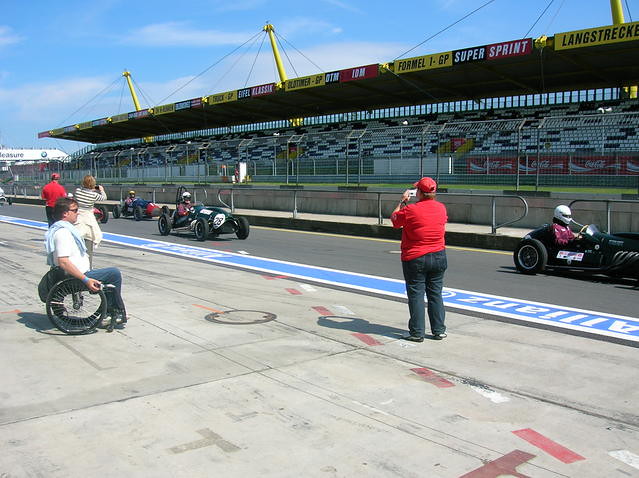The photograph captures a dynamic scene at a racetrack with a light blue sky dotted with various white clouds overhead. Multiple small, tubular race cars with black tires and silver rims speed from left to right across the black asphalt track, which features yellow lines on the outer edge and a blue banner with white borders and lettering on the inner edge. In the background, the audience seating area, filled with white and black folding seats and covered by a canopy, is separated from the track by a green field and a fence. The scene also includes various spectators: a man in a wheelchair wearing jeans, a white t-shirt, sunglasses, and a scarf-like accessory, and a woman in dark jeans, a red t-shirt, and a red baseball cap, who is holding a camera with her back turned to the viewer. Another detail of the setting is the flat pavement area in the foreground where people are positioned, capturing the excitement of the race.